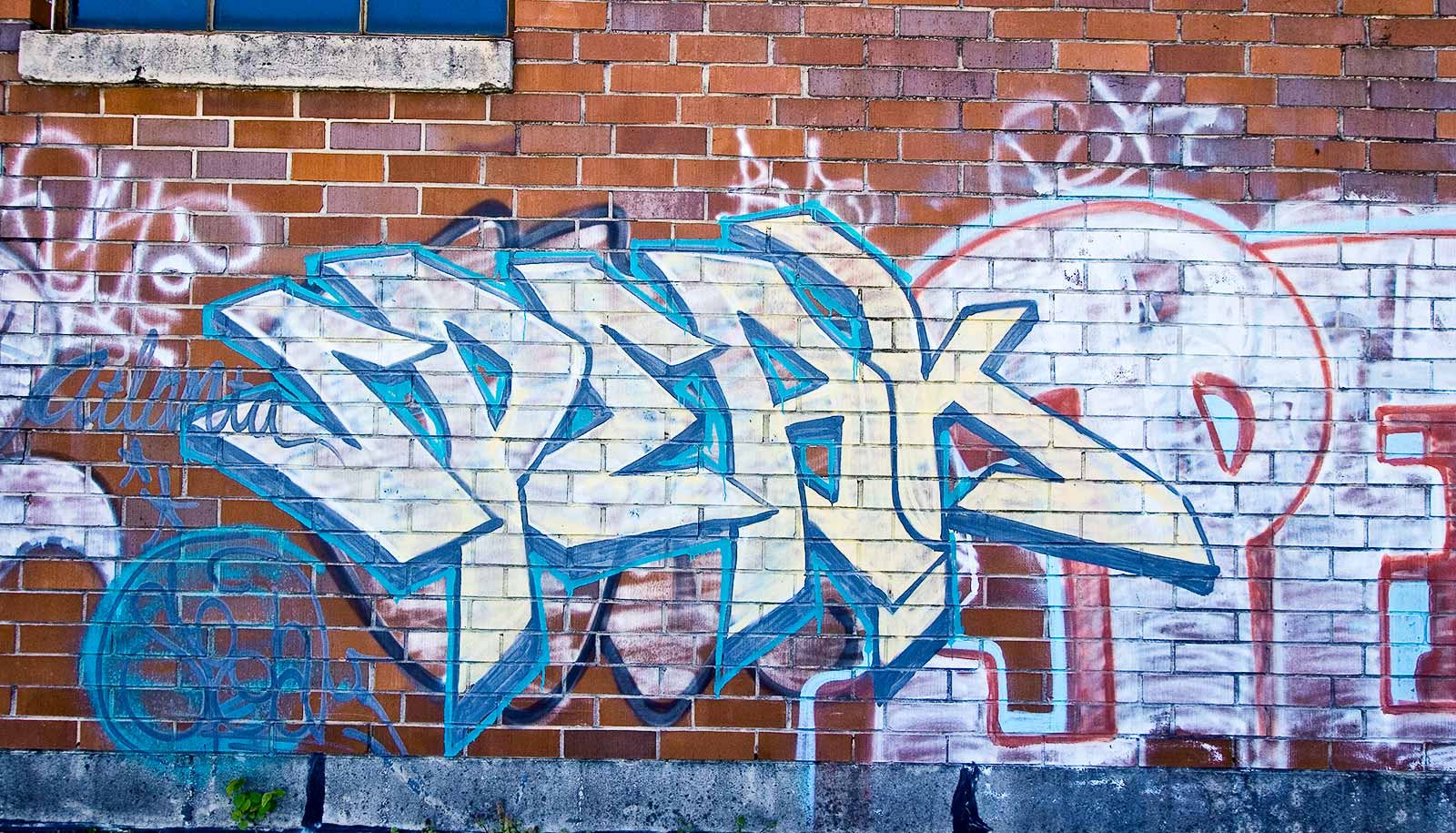The image depicts an expansive red brick wall extensively covered in graffiti. The bricks predominantly exhibit orange and red hues, with the left-hand side showing fairly recent white masonry and the right-hand side displaying older, cracked mortar. In the upper left corner, part of a concrete window lintel extends out of the frame, while the top right reveals remnants of a blue window and a window sill built into the wall. The central focus of the graffiti is the word "speak," rendered in large, stylized white and yellow letters with a blue shadow effect, giving it a three-dimensional appearance. Surrounding this dominant piece, additional graffiti in various colors, including blue, white, and red, can be seen, although much of it is illegible. The word "boys," spelled "B-O-Y-Z," and the word "Atlanta" in blue script accompanied by two stars are also visible amidst the chaotic spray-painted artwork. At the base of the wall, gray stone rectangles replace the typical red bricks.